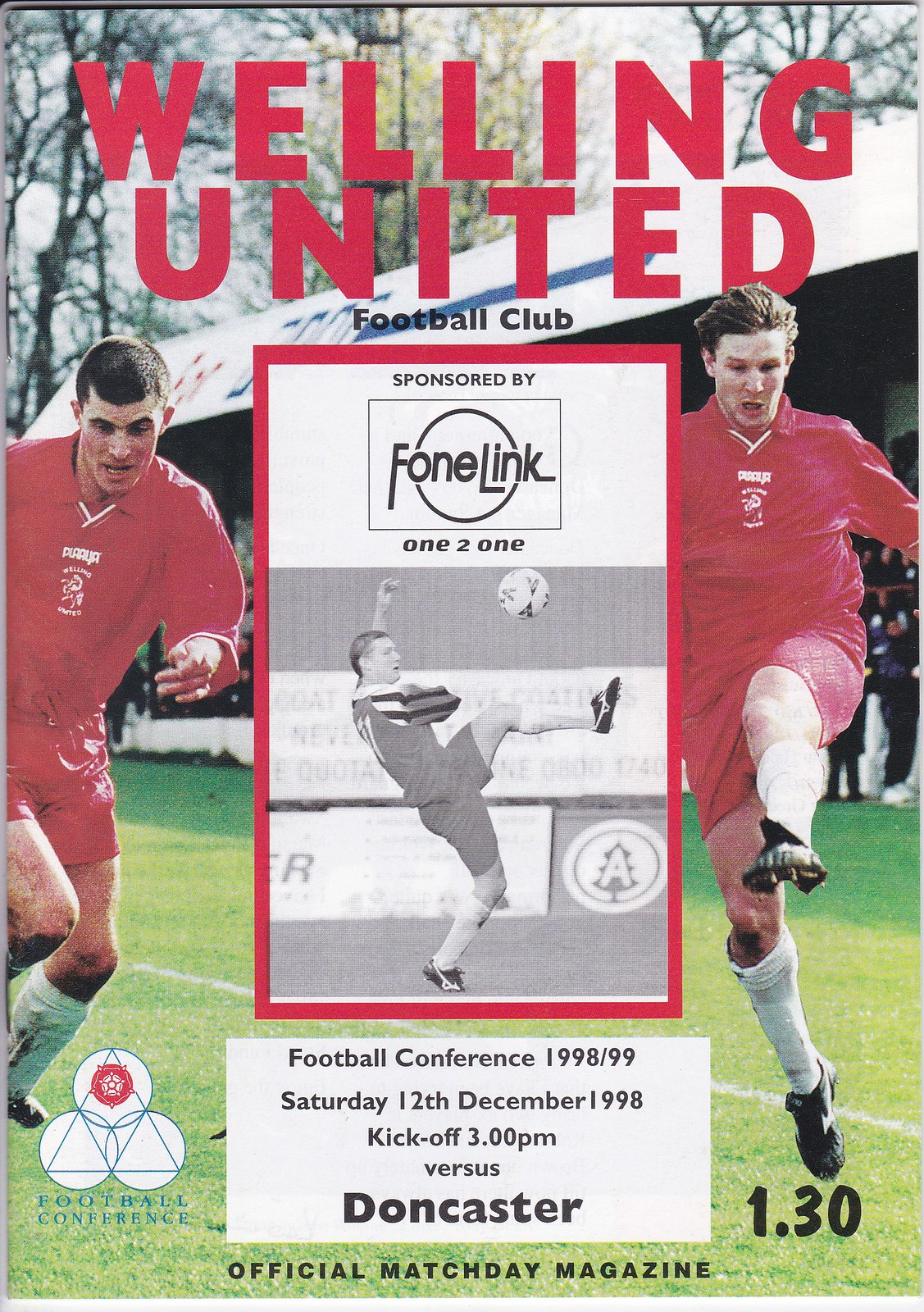The cover of the magazine showcases a bright spring day scene from a Welling United Football Club match. At the top of the cover, "Welling United Football Club" is written in bold red letters. Below this, there are two players dressed in red uniforms with white socks and black shoes, captured in action as they concentrate on the game, kicking a soccer ball across the green field. The background features stands and barren trees. In the middle of the cover, there's a black-and-white picture of another soccer player, mid-action with his right leg extended and a soccer ball hovering above it. This image is accompanied by a sponsorship notice saying "Sponsored by Phone Link" in red. Further down, within a white box and black print, details about the match are provided: "Football Conference 1998-1999, Saturday, 12 December 1998, kickoff 3 p.m. versus Doncaster." At the very bottom, it notes "Official Match Day Magazine." Additionally, beneath the player on the left, there's a formation of three soccer balls, creating a triangular shape, with the top ball featuring a red dot in the center. The figure "1.30" is inscribed on the grass.